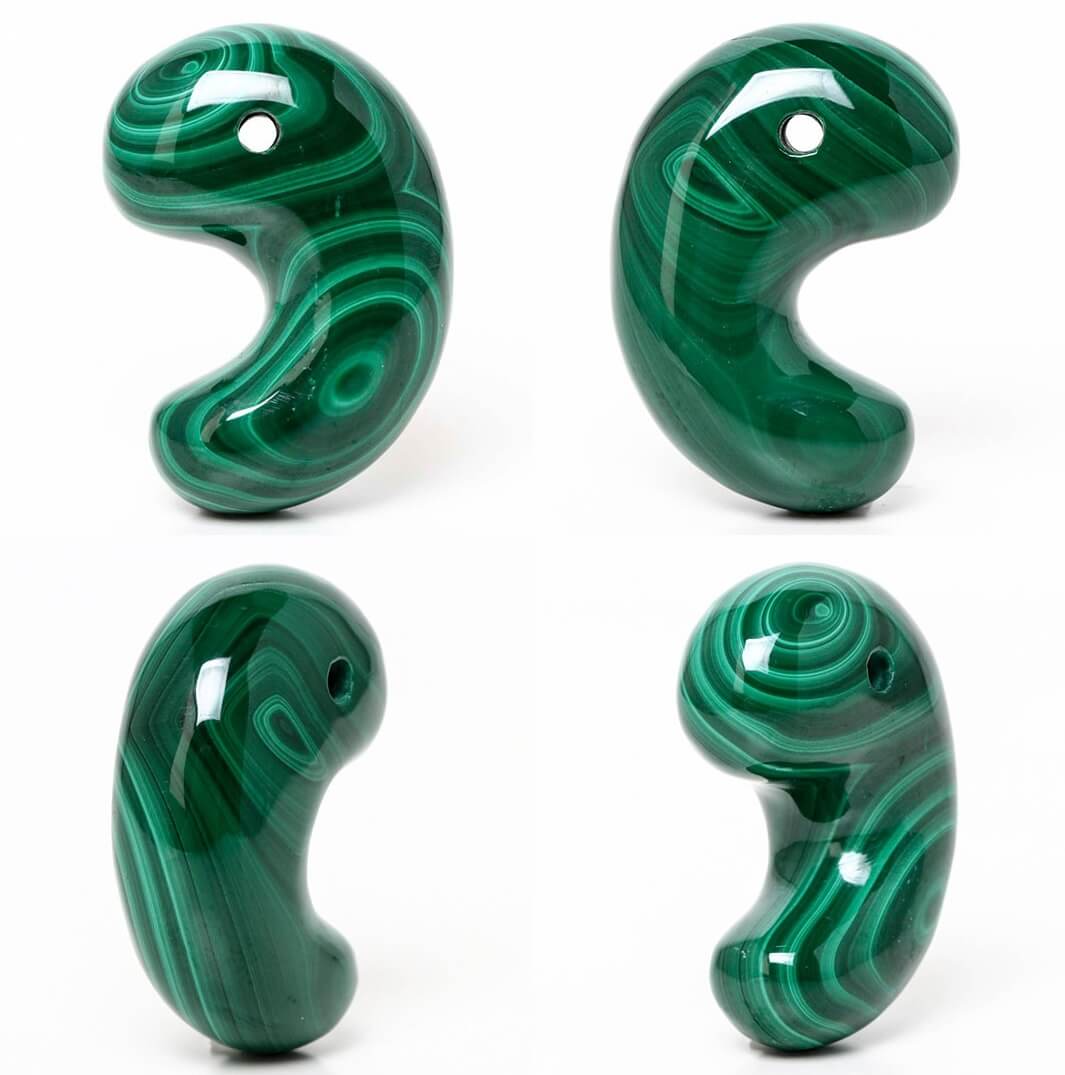The image presents four highly polished, green glass sculptures arranged on a stark white background. Each sculpture is C-shaped, somewhat reminiscent of a tadpole or a decorative earpiece, and features a hole near the top, adding an eye-like appearance. The sculptures are made from a green glass material with darker green interiors and lighter green, concentric ring patterns that resemble the swirling clouds of Jupiter or Saturn. Each figure is glossy and reflective, marbled with intricate, white, cloud-like designs. The four sculptures are displayed in quadrants: the upper left sculpture faces left, the upper right faces right, the lower left is viewed from a backward angle, and the lower right faces forward, slightly turned left. The detailed craftsmanship and polished surface give them a unique, elegant appearance, almost like carved, decorative green beans or the insides of a geode.